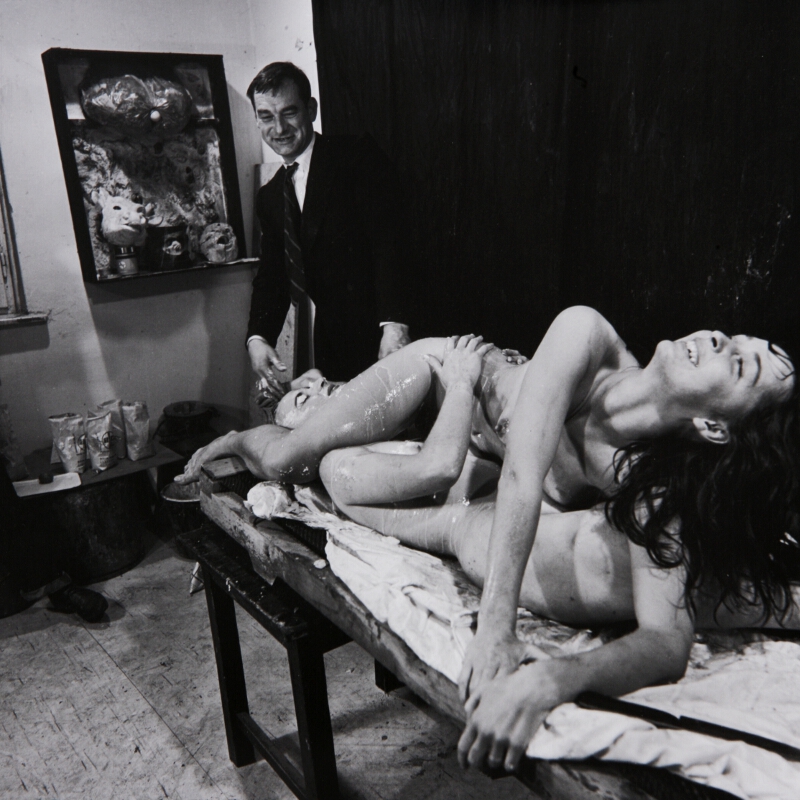In this evocative black-and-white photograph, a scene of performance art or erotic display unfolds in the corner of a room. The right-hand wall is draped with black curtains while the left-hand wall is stark white, creating a contrasting backdrop. Central to the image is a makeshift table, resembling a thin mattress propped up on a stool. On this mattress lies a man on his back, with his legs extending from the right side of the photo towards the center. Positioned atop him, oriented in the opposite direction, is a woman with long dark hair, her legs near his upper body and her head near his lower body. She twists her torso to look upward, eyes closed, mouth open in a smile.

Both individuals appear nearly naked, save for parts of their bodies wrapped in transparent saran wrap, giving a translucent, wrapped effect. A third figure stands beside them—another man dressed in a dark suit jacket, striped tie, and white shirt. His short dark hair frames a face looking down at the pair with a faint smile. Scattered around are objects like soda cups and a shelf with small statues, along with a table cluttered with packets, contributing to the cluttered, yet intimate ambiance. This intricate tableau, captured in monochrome, exudes an enigmatic blend of vulnerability and voyeurism.